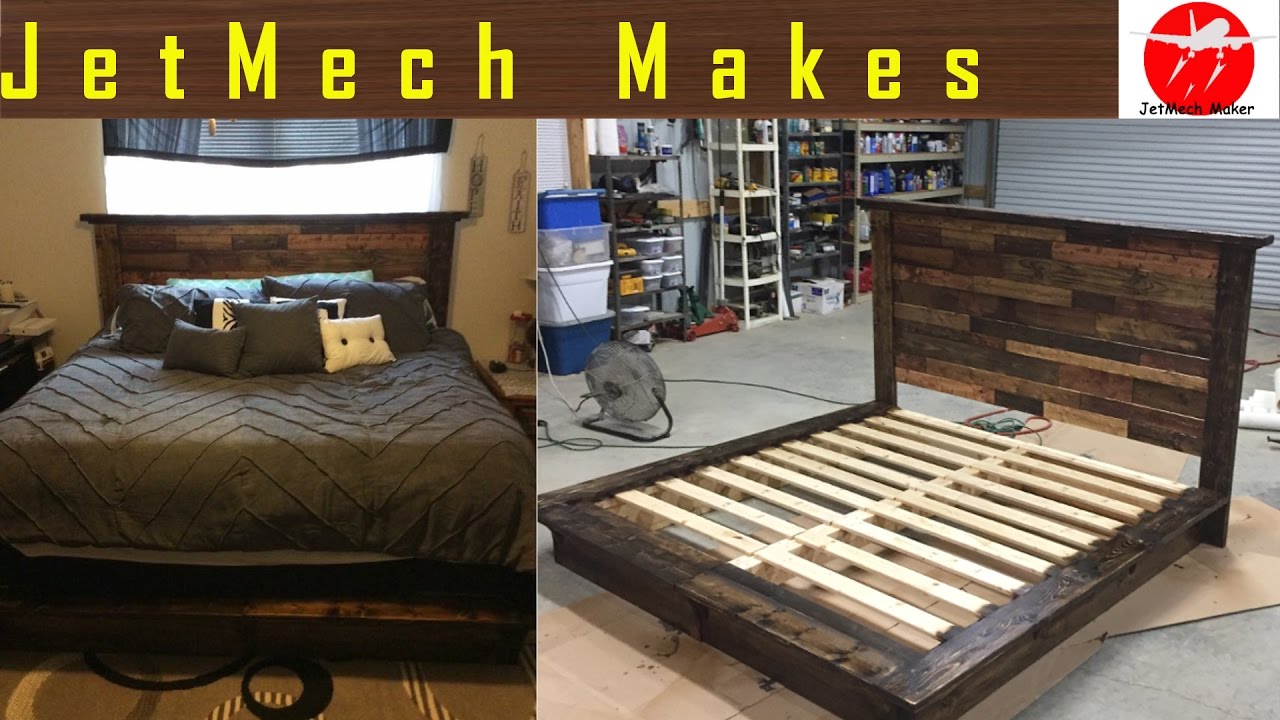This photograph appears to be an advertisement for Jet Mech Makes, showcasing a bed frame in two stages. At the top, bold yellow text on a brown banner reads "Jet Mech Makes." In the upper right corner, there's a logo featuring a gray jet within a red circle, labeled "Jet Mech Maker" in black Comic Sans font.

The image is divided into two panels. The left panel depicts a fully furnished bedroom with a bed made up of a dark wood headboard and frame. The bed is neatly dressed with a dark chocolate comforter, multiple pillows in various shades of brown and cream, and a single white pillow. Above the bed, there’s a window partially covered by a dark blue shade, with nightstands flanking the sides.

The right panel shows the bed frame in what appears to be a workshop or garage. The unfinished frame features a headboard with multiple shades of wood arranged horizontally and light tan wooden slats running lengthwise to support the mattress. The workspace is cluttered with tools, storage shelves, a saw, and a small fan on the floor. This dual-image setup highlights both the craftsmanship and the final product, emphasizing the manufacturing process and the finished, assembled bed.